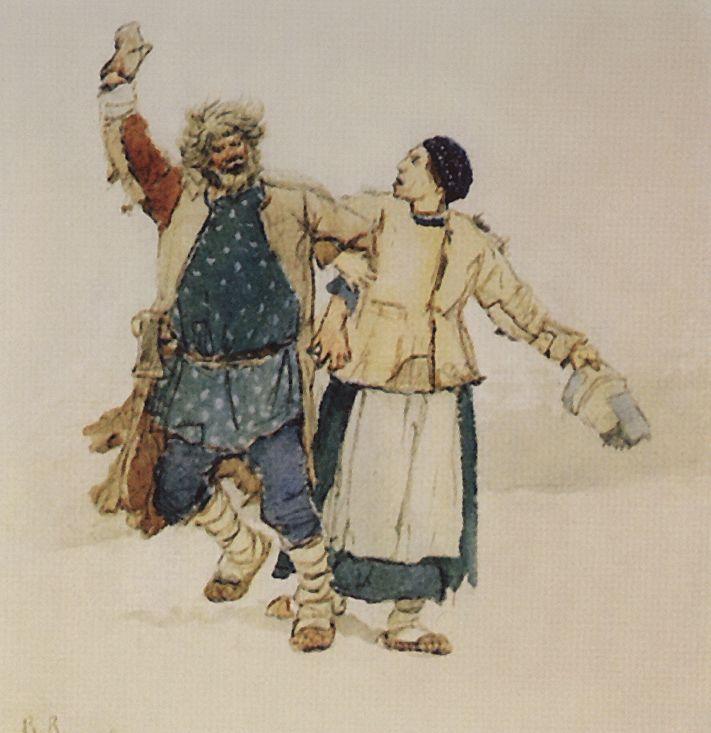This painting, reminiscent of an advertisement, depicts an older man and woman, possibly peasants from a historical era. The man exudes a joyful and vibrant energy, reminiscent of Santa Claus, with his white beard and hair, and a red jacket with a white collar. However, there are some variations in each description, suggesting his robust form is adorned in a sheepskin or animal skin-like beige tunic extending past his knees, paired with a rope belt and blue pants that end at the mid-calf. His feet are protected by white leggings wrapped with rope to secure them. He raises his right arm joyfully with his right foot off the ground, hinting at a dance step, perhaps suggesting a lively moment caught in time.

The woman, arm-in-arm with the man, appears to be his wife. She seems to be leading or supporting him, maybe even sharing in the dance, though her expression ranges from annoyed to singing. Dressed in a long blue dress and a white apron, partially covered by a cream-colored smock or jacket, she too wears fabric or animal skin shoes and white tied leggings. Her hair is tied back, and she dons a knit hat. Her left hand is holding an indistinct object, possibly his hat, further emphasizing their interaction.

The shared background in all observations is relatively bare, with a cream hue, ensuring the focus remains on this vibrant couple. Their weathered and well-worn attire suggests a simpler, rustic lifestyle, adding a touch of historical authenticity and perhaps humor to their portrayal.